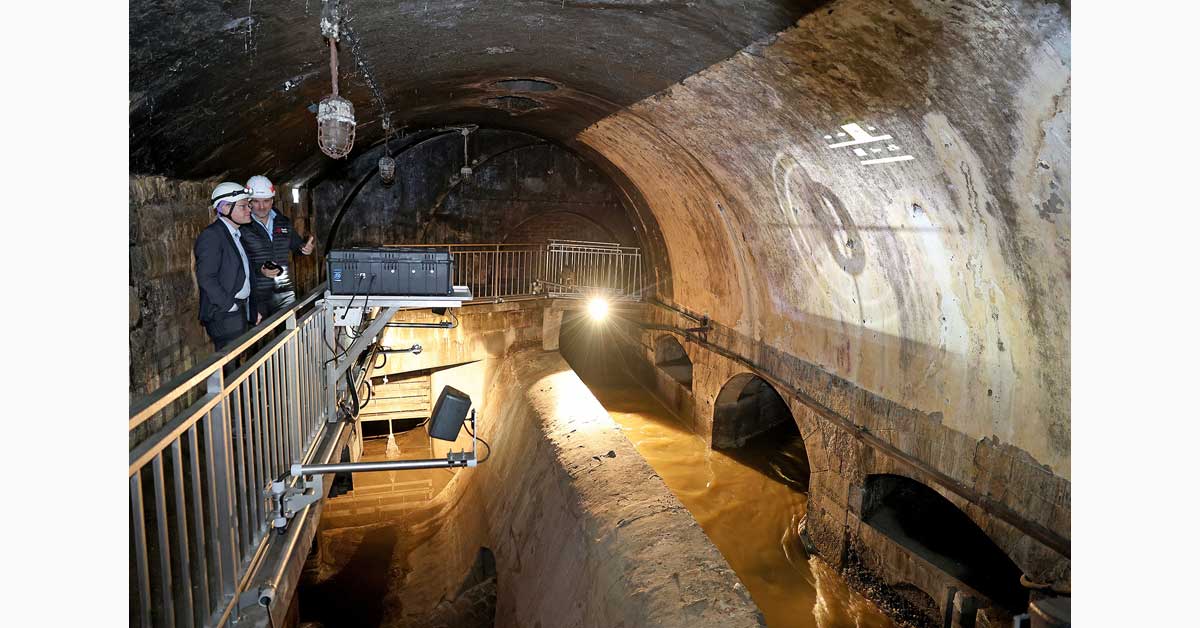The image depicts the interior of a tunnel-like structure, possibly part of a manufacturing plant or a dam where water flows. In the left side of the image, two men stand behind silver railings. Both men are dressed in blue jackets with light-colored shirts underneath and are wearing white helmets, one of which is equipped with lights. The man on the left, who appears to be in conversation, has both hands raised, while the man on the right has his right hand in his pocket. He also wears glasses and holds a flashlight. The tunnel itself is constructed of brownish-gray material with water visible at the bottom. Overhead, several lights illuminate the space, and there are multiple smaller sub-tunnels or culverts visible at the bottom. The scene is further detailed by a large, bright yellowish-white light in the center of the photo, and another silver railing can be seen in the background. Additionally, a black box with a wire and a toolbox are present, suggesting an industrial setting.